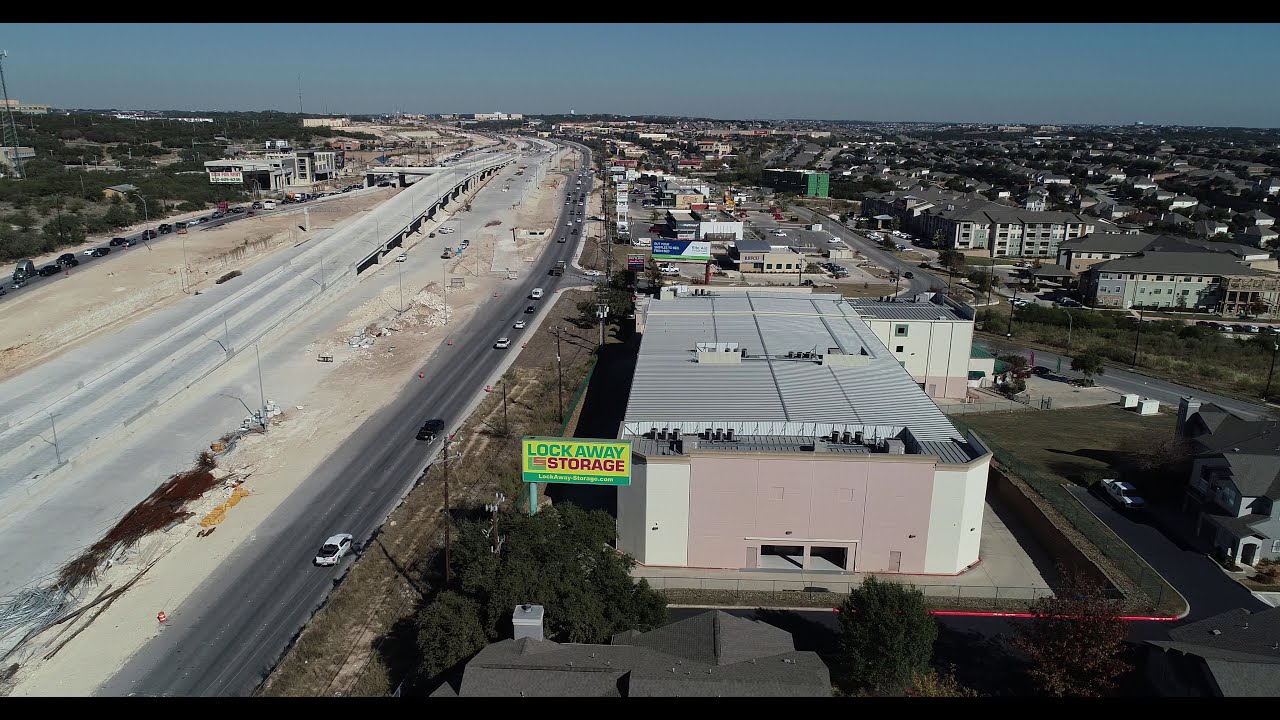The photograph, taken from above using a drone, captures a commercial area in what appears to be a small city or large town. The image is in color and is oriented in landscape format, showcasing a varied urban layout. On the left side, two paved roadways run in parallel from the bottom edge to the top center, one of which curves and disappears into the horizon. Adjacent to these roads, a bridge crosses over another road, flanked by patches of dirt, suggesting construction activity. A dirt "sand island" is also visible to the left of the main highway.

To the right of these roads, the foreground features a large, rectangular building with a light pink stucco wall, which houses a storage facility named "Lockaway Storage." The sign for this facility is prominently displayed on the top left of the building, with 'Lockaway' written in green letters and 'Storage' in red letters, set against a yellow background. Behind the storage unit is a parking lot, and further north are clusters of corporate buildings and potentially motel-like structures, with several smaller roads running between them.

In the backdrop, the sky is a clear blue, devoid of clouds, adding a serene contrast to the busy commercial scene below. A billboard is also present behind the buildings, although its text is not discernible. This high-angle, realistic photograph effectively captures the intricate details of the business warehouse district, with its various commercial buildings, motels, and intersecting roads.